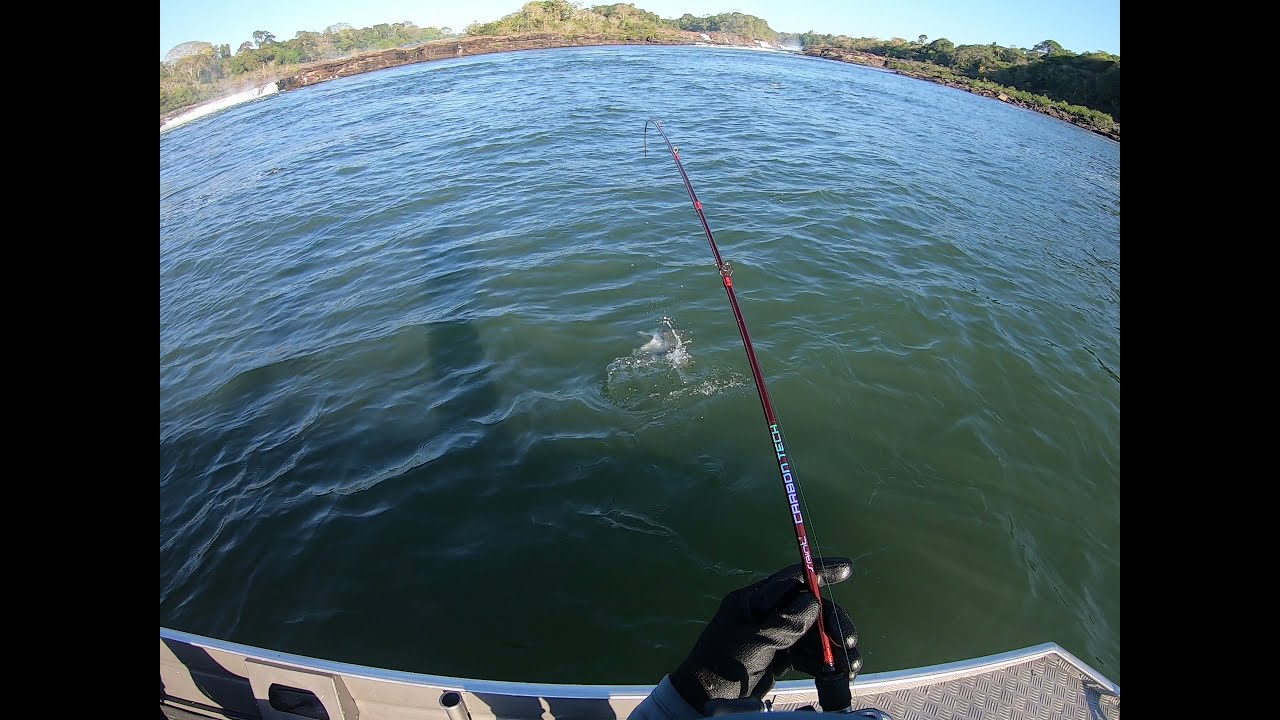The photograph captures an angler's perspective from a light gray boat on a green, murky lake or river with vegetation and possibly a small beach in the distance. The fisherman, wearing black gloves, holds a red fishing rod with blue detailing and faint white lettering, and the rod is visibly bowed, indicating a significant catch just below the water's surface. The surroundings feature different shades of gray, black, red, white, green, tan, and brown, with water occupying the majority of the image, flanked by land at the top. The scene is set on a bright, clear day, showcasing greenery and a blue sky, suggesting an outdoor fishing adventure in a tranquil, natural setting.